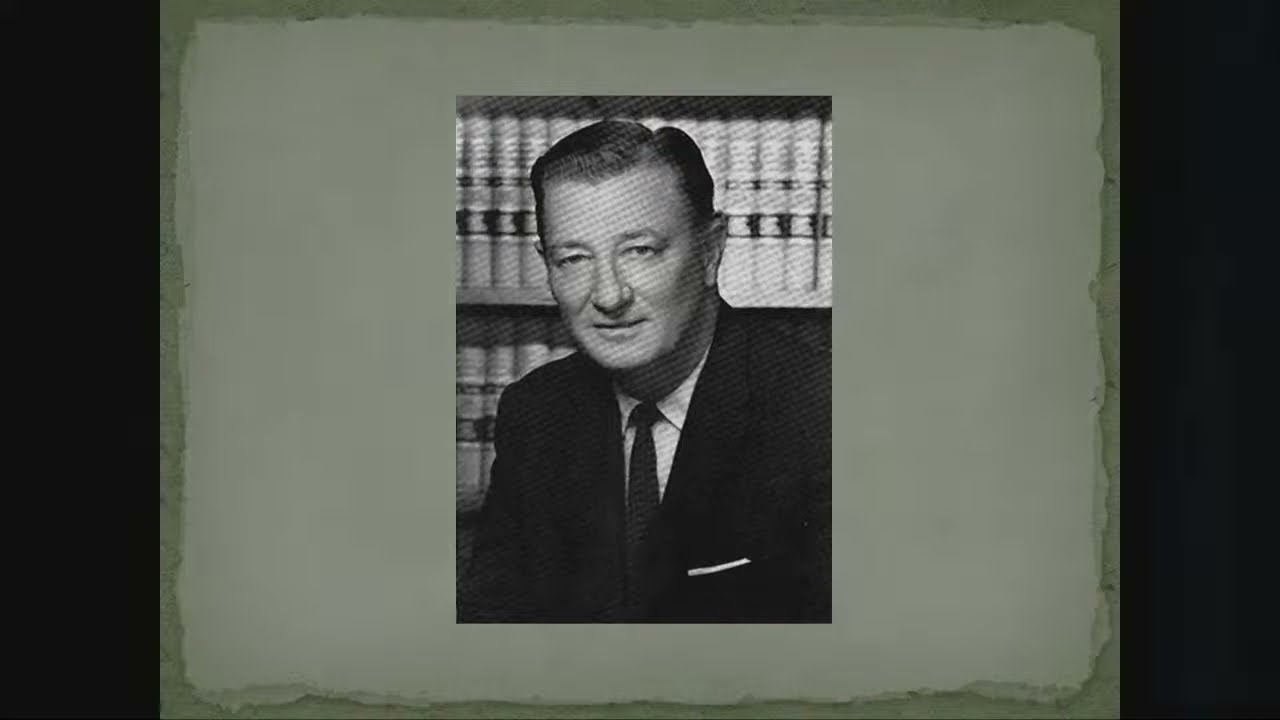A photograph depicts a heavyset, bald man of indeterminate race, standing behind a black lectern during a presentation. He is gesturing animatedly with one hand raised while the other rests on an open book atop the lectern. The man is wearing glasses with black frames and sports a short beard and mustache. His attire includes a black blazer over a light blue and white checkered button-down shirt. He also has a microphone clipped to his shirt. The background is predominantly black, with a neon blue light illuminating the left side of the image. A black microphone is visible to the man's left, emphasizing his role as a speaker in this setting.